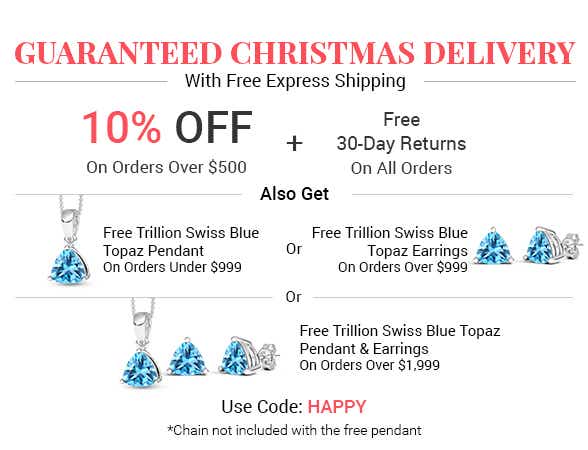**Guaranteed Christmas Delivery!**

*With Free Express Shipping*

---

**10% OFF**  
*on orders over $500*

---

**Free 30-day returns on all orders**

---

**Also Get:**

- **Free Trillions Swiss Blue Topaz Pendant** (on orders under $999)
- **Free Trillions Swiss Blue Topaz Earrings** (on orders over $999)

---

**OR**

**Free Trillions Swiss Blue Topaz Pendant and Earrings** (on orders over $1,999)

---

**Use code HAPPY** (in all caps, written in red)

**Note:** *Chain not included with the free pendant.*

---

Images of the Trillions Swiss Blue Topaz Pendant, Earrings, and Pendant & Earrings Set (all set in what looks like silver).